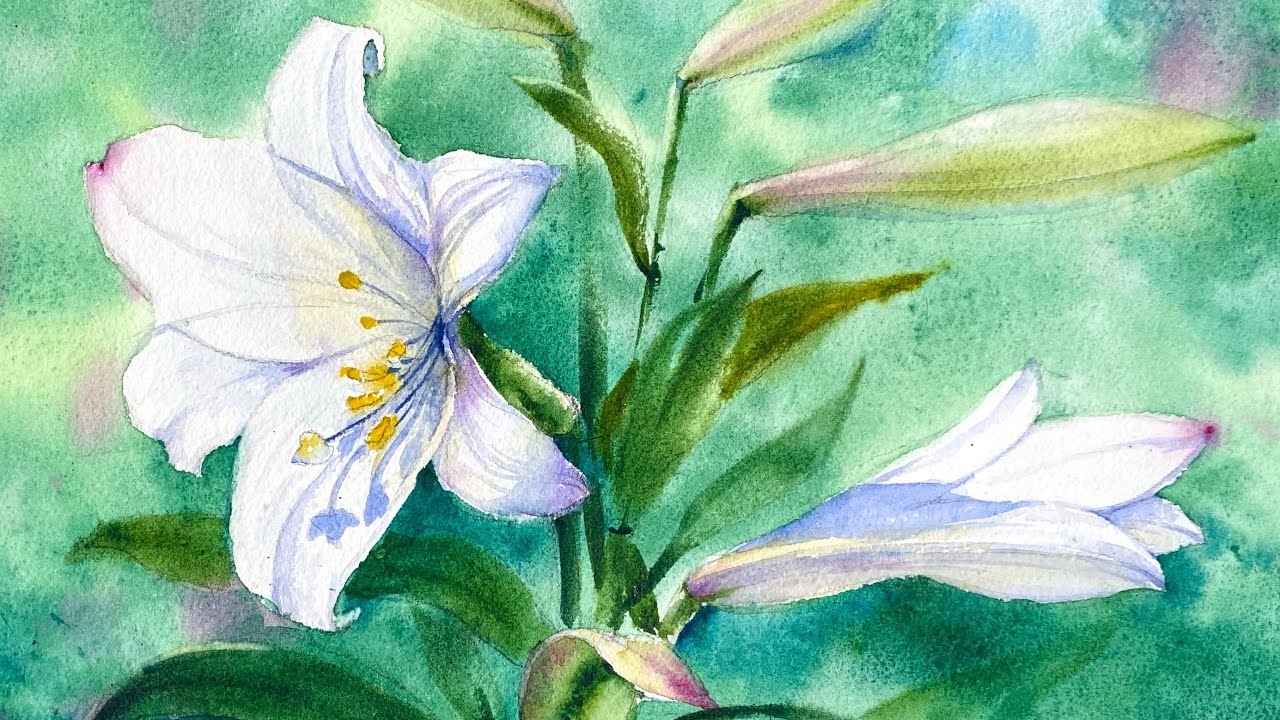This image shows a highly detailed watercolor painting of a flower arrangement, captured in a photograph. It features two main flowers on a backdrop of soft, blotchy greens, creams, blues, and pinks. The focal point of the painting is a large white flower on the left, characterized by six elongated oval-shaped petals with tapered points, one of which has a red tip, and showcasing vibrant yellow stamen at its center. Accenting the white petals are hints of blue, adding depth to the painting. To the right, a tall, green stem supports a second, not-yet-bloomed white and blue flower with a pink tip, portraying a sense of growth and anticipation. Interspersed among the flowers are elliptical green buds, indicating future blossoms and adding to the painting’s dynamic composition. The background’s soft focus emphasizes the flowers' vivid details, creating a harmonious blend of nature’s colors and forms.